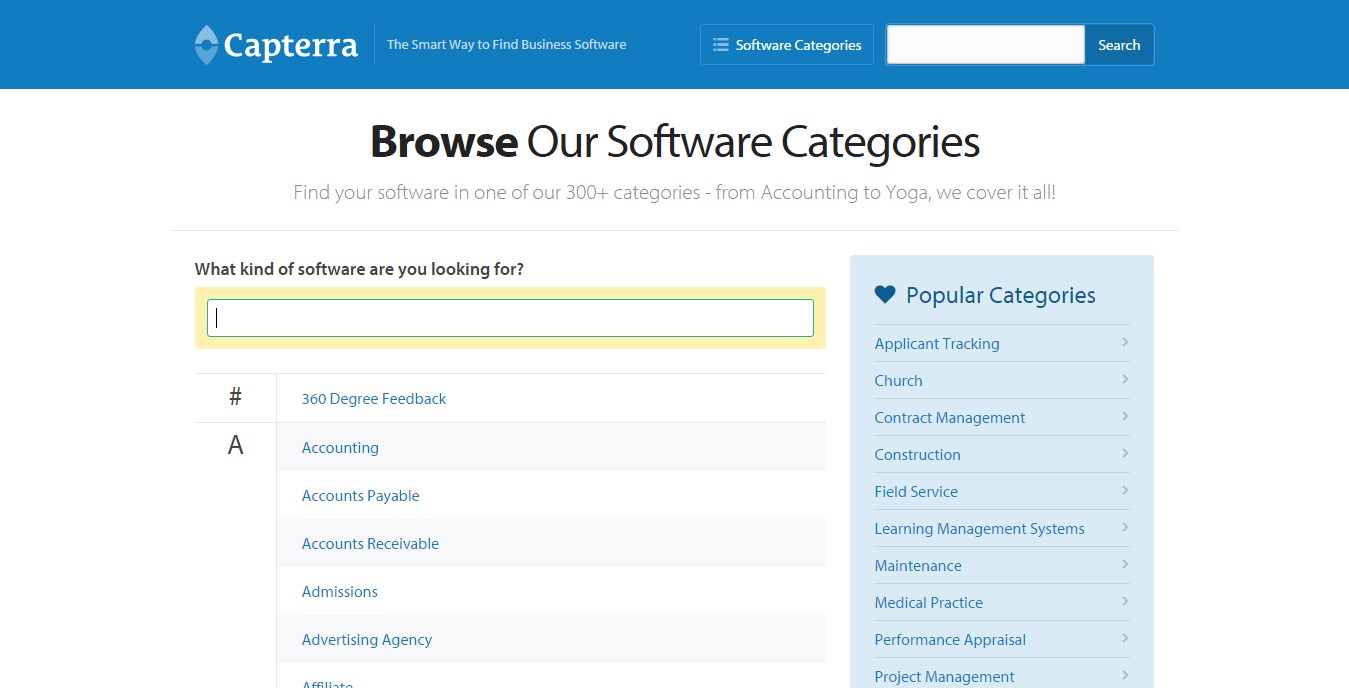This is a screenshot of the Captira website. At the top of the page, a blue navigation bar stretches across the width of the site, prominently displaying the website's name "Captira" along with its logo on the left side. Located near the logo are up and down arrow icons. On the far right side of the blue bar, there's a tagline that reads "The smart way to find business software." Below this tagline, a white box with a white outline contains the phrase "Software Categories," which is positioned next to a search bar. The central section of the page features a heading that says "Browse Our Software Categories" followed by an invitation to "Find your software in one of our 300+ categories, from accounting to yoga—we cover it all." Beneath this heading, another search bar outlined in yellow prompts users with the message, "What kind of software are you looking for?" The overall layout is aimed at helping users easily find and navigate through various software categories.